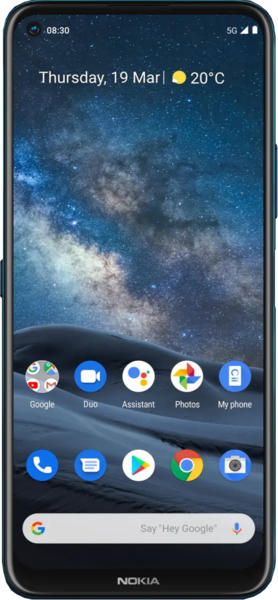This image showcases a sleek black Nokia Android device. However, the power button on the upper right edge has a light blue hue, suggesting a possible dual-tone exterior. The display wallpaper features a stunning galaxy theme, with a blue sky dotted with white stars and adorned with several gray clouds. At the bottom of the wallpaper, there appears to be some atmospheric land in shades of gray and blue.

The interface displays essential information: at the top, in white text, it reads "Thursday, 19 Mar" with a divider line below it. Underneath, a yellow sun icon with some clouds indicates the weather as 20 degrees Celsius. The current time, "08:30," is prominently displayed in white on the top left. On the right, the status bar shows the 5G network with full signal strength and a fully charged battery icon.

The bottom of the screen is populated with various application icons arranged in a circular format. From left to right, these include a Google Apps subfolder, Duo, Assistant, Google Photos, My Phone, a blue caller button with a white phone icon, Messages, Play Store, Google Chrome, and a camera icon. Below this row of icons, there's a large oval area in white. On the left side of the oval is the Google "G" symbol, while the right side features the text "Say 'Hey Google'" in gray Arial font, accompanied by a microphone symbol in Google colors.